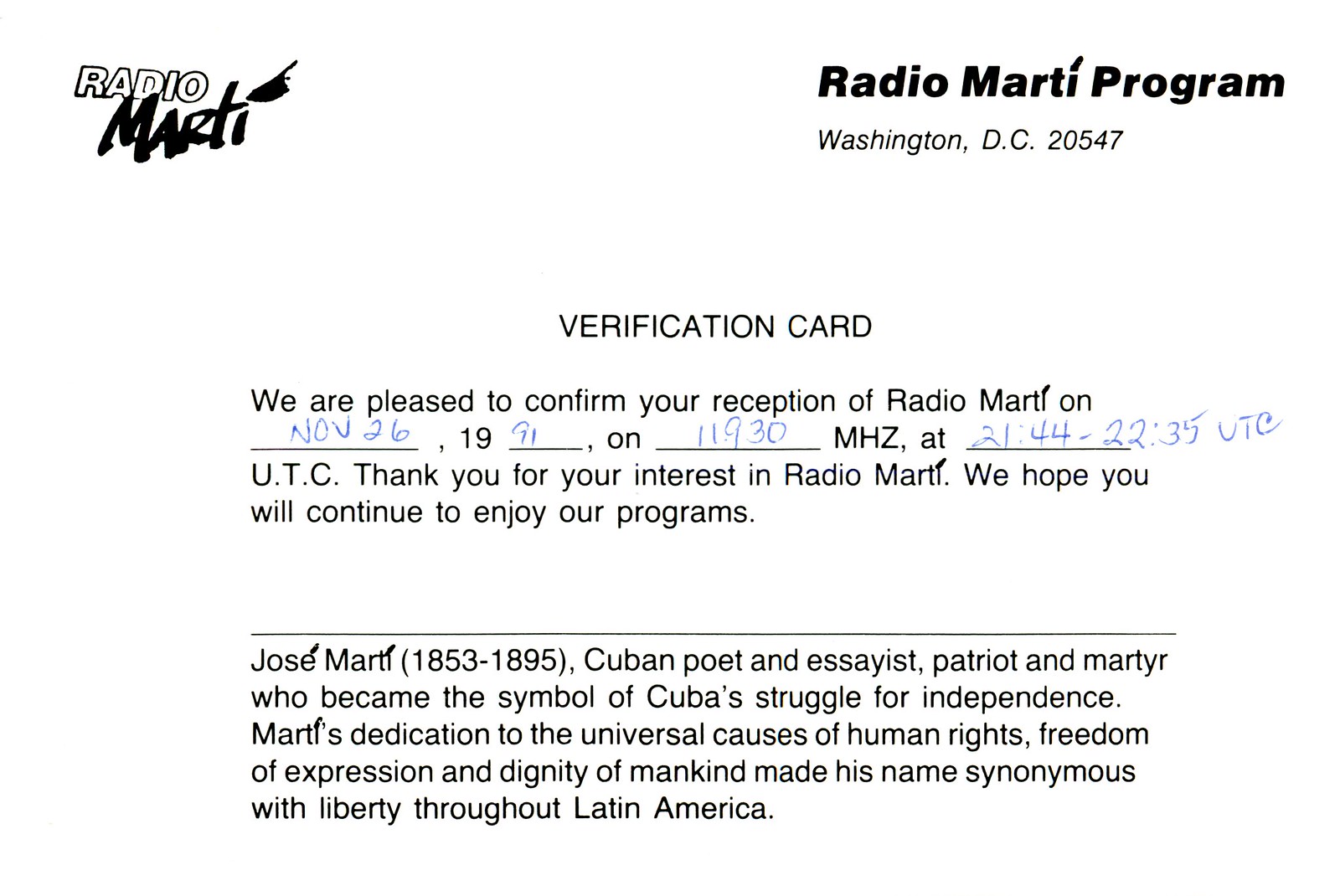This photograph features a black and white verification card from Radio Marti. In the top left corner, it reads "Radio Marti, M-A-R-T-I," and on the top right, it states "Radio Marti Program, Washington, D.C. 20547" as the letterhead. Centered on the card in capital letters is the phrase "Verification Card." The text below confirms the reception of Radio Marti on November 26, 1991, at 11930 MHz at 0445 UTC, expressing gratitude for the listener's interest in Radio Marti and hope that they continue to enjoy their programs. A solid black line separates this information from a tribute to Jose Marti at the bottom. It notes that Jose Marti (1853-1895) was a Cuban poet and essayist, patriot, and martyr who became a symbol of Cuba's struggle for independence. His dedication to the universal causes of human rights, freedom of expression, and the dignity of mankind made his name synonymous with liberty throughout Latin America.